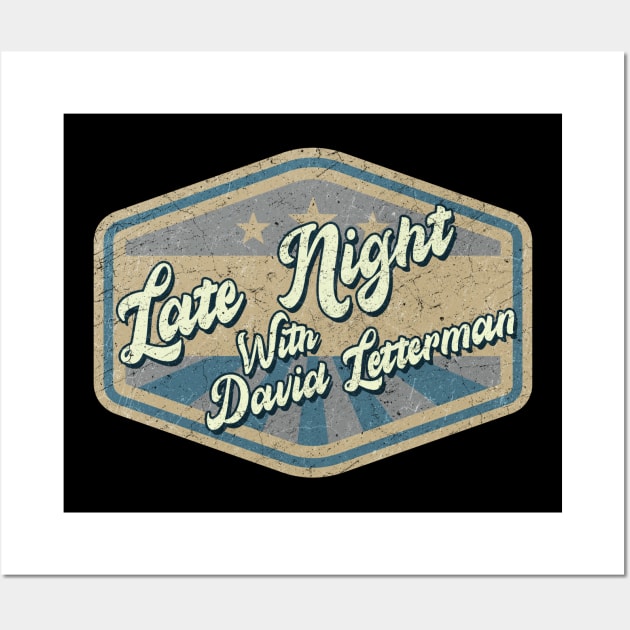The image displays a promotional banner reminiscent of a vintage commercial advertisement. It has a horizontally rectangular shape with a light gray border at the top and bottom, and a white border encasing the entire sign. The predominant background is a solid black, which accentuates the focal sign in the center. This sign features a six-sided shape with a light tan and light blue color scheme, reminiscent of a coat hanger, filled with alternating light and medium blue stripes. Additionally, there are three white stars on the blue section of the sign, giving it a somewhat patriotic feel despite its faded and cracked design.

The text on the sign reads "Late Night with David Letterman" in white cursive letters with a shadow effect, each word's initial letter capitalized. The stark contrast between the white text and the black background ensures the message stands out clearly. There are no other texts or numbers present, and the image is devoid of any people. Its high clarity and absence of distortion make the details easily discernible. The overall ambiance of the image is bright, maintained by ample natural light, effectively highlighting the sign without any blurriness.